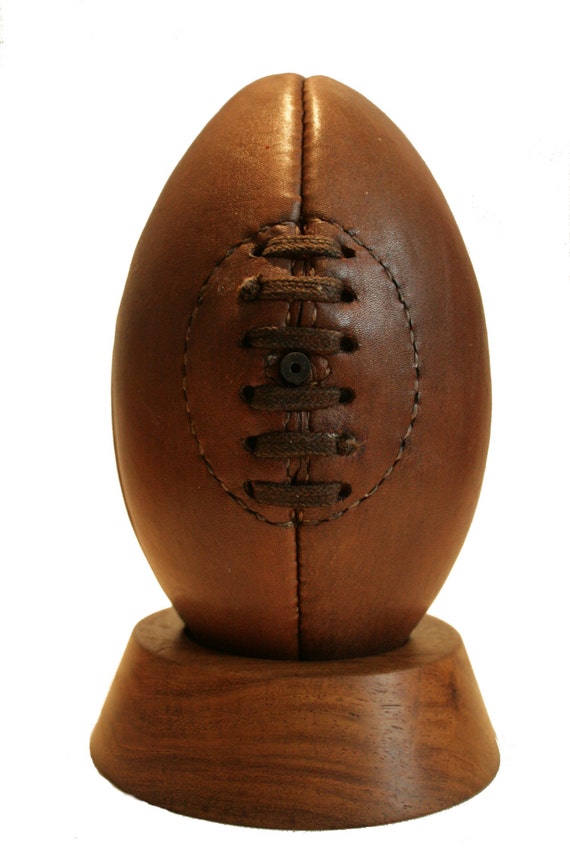The image showcases a vintage American football, prominently made from leather and showcasing an aged appearance. This brown, egg-shaped football features distinct laces resembling shoestrings, threaded through 12 holes, which securely connect both sides of the ball. A small inflation vent is noticeable in the center. This beautifully aged football is carefully displayed on a sturdy, dark wooden stand that matches the football's hue. The stand, approximately two to three inches tall, has a specifically designed indentation to hold the football upright. The setting of the image appears to be a museum display, with the football and stand placed against a plain, white background, emphasizing the historical and pristine nature of the exhibit.